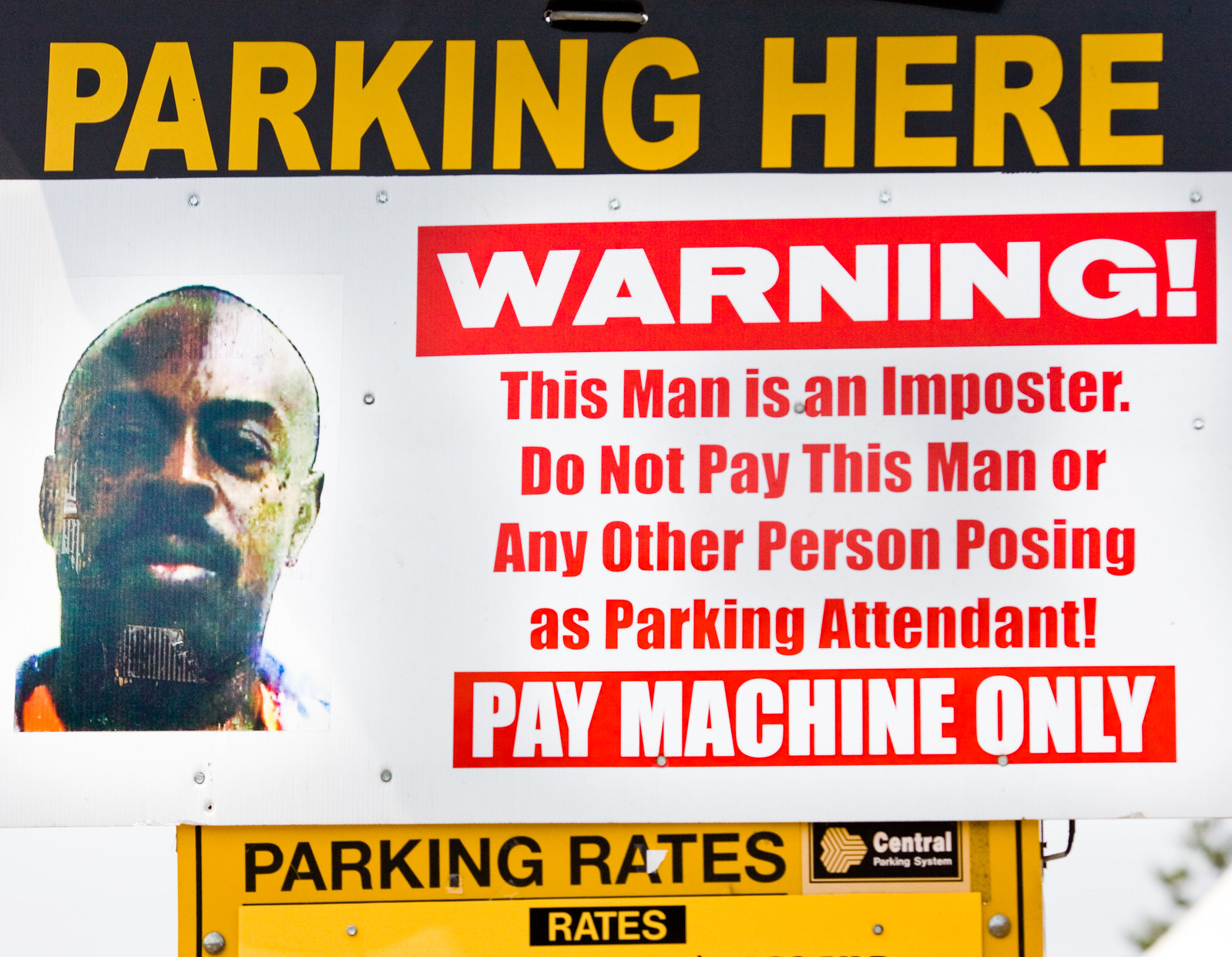This is a detailed color photograph of a close-up warning poster attached to a parking rates sign from Central Parking Systems. The poster features a headshot of an African American male wearing a black and orange jacket. The man, who is bald and has a stubble beard, is staring directly at the camera. The poster prominently displays very large, bright text on a black background reading "PARKING HERE." Below this is a stark warning in red letters on a white background: "WARNING: THIS MAN IS AN IMPOSTER. DO NOT PAY THIS MAN OR ANY OTHER PERSON POSING AS PARKING ATTENDANT. PAY MACHINE ONLY." The entire poster is visibly stapled to the sign, which also lists the parking rates.